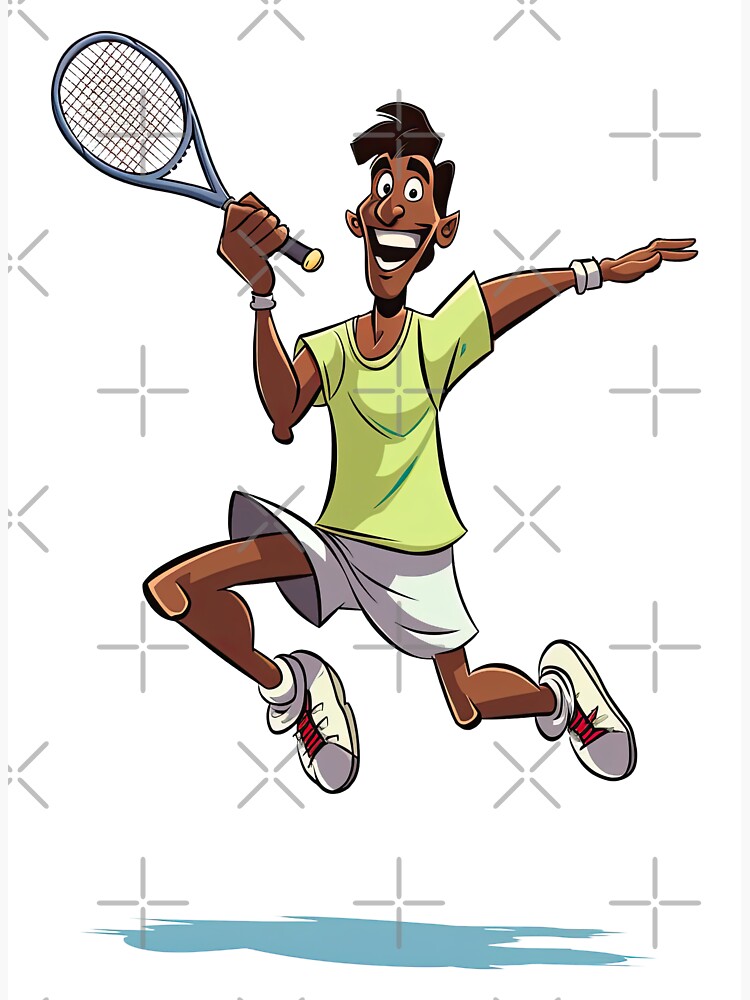The cartoon image features an exuberant man with dark brown skin and short, dark hair, possibly of African-American or Indian descent. He is depicted mid-jump on a white background with a light teal-blue shadow cast below him. The man is wearing white shorts, white tennis shoes with red laces, white socks, and white wristbands, complemented by a lime green-yellow t-shirt. His expression radiates joy and excitement; his wide-open mouth reveals large white teeth, his eyebrows are raised, and his eyes are round and expressive. In his right hand, he holds a tennis racket with a dark blue frame and gray strings, while his left arm extends outward at his side. He appears clean-shaven and full of energy, with his knees bent and both legs off the ground, clearly engrossed in the spirited activity of playing tennis.